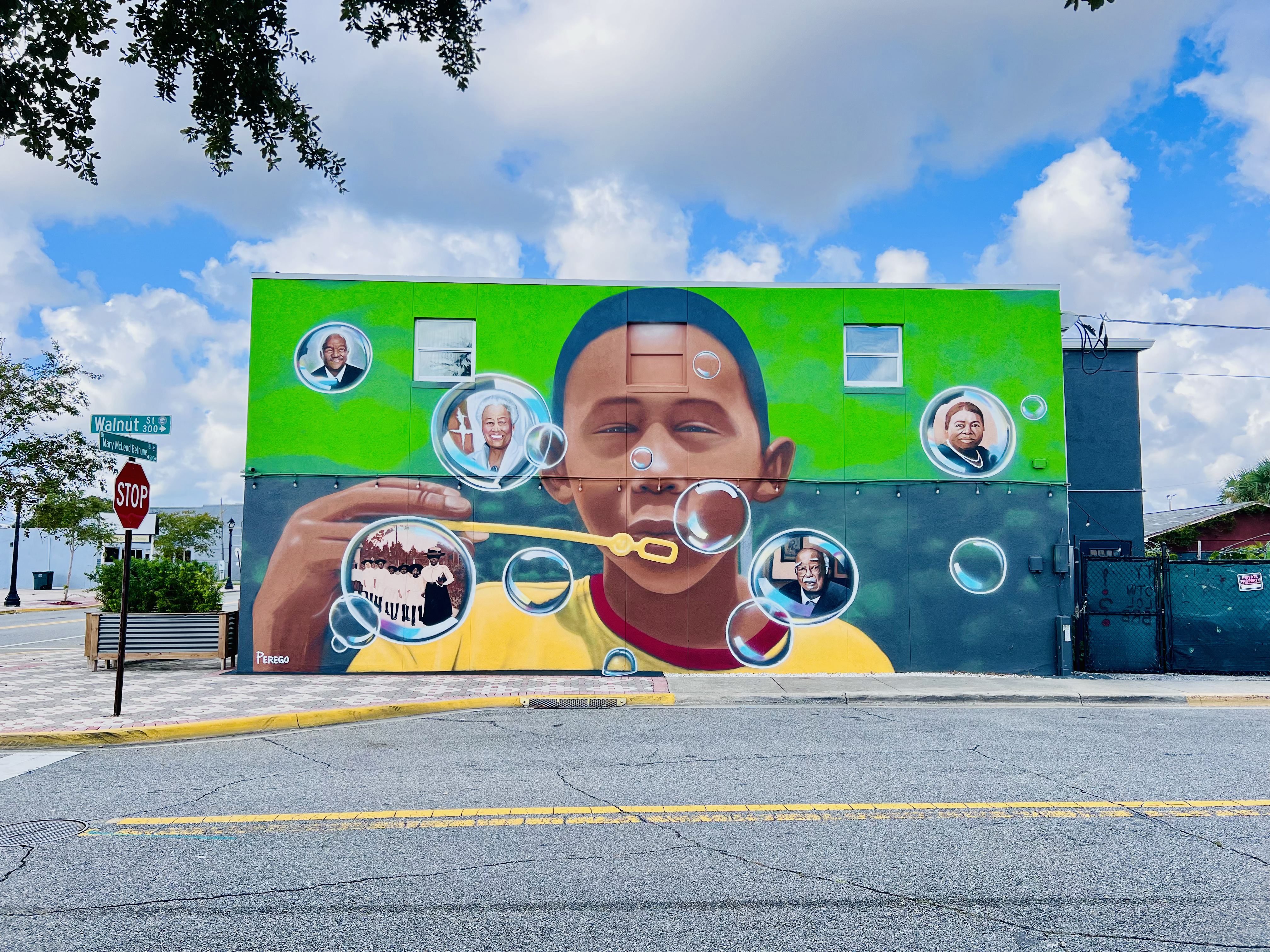The image captures a vibrant and detailed street scene focusing on an intricately painted mural on the side of a rectangular, horizontally-oriented building. This outdoor wall mural, viewed from across the street in a color photograph, features a young African-American boy, approximately nine years old, with short black hair and eyes closed, holding a yellow wand to blow bubbles. He is depicted wearing a bright yellow shirt with a red ring around the neck, and the mural shows him from the top of his head to his shoulders.

The mural is divided into two main color sections: the top half showcases a bright green band and the bottom half features a denim blue band. Adding to the colorful scene, the sky above the mural is a clear blue with white clouds. Around the boy, there are several bright white bubbles, each bubble having detailed faces within them. In particular, the upper left and middle bubbles contain portraits of older, apparently respected community figures, while the lower left bubble shows a vintage black-and-white photograph of a teacher with children. On the bottom right, another bubble contains the image of an elderly black man dressed in a suit with a white mustache.

The building also features two square windows at the top of its second story, blending seamlessly into the mural. The street below includes a sidewalk, a stop sign, and several trees, while adjacent buildings and a bench can be seen further to the right, enhancing the realism and communal atmosphere of the scene. The style of the mural is photographic representationalism realism, making the artwork stand out with its vivid colors and detailed portraits.